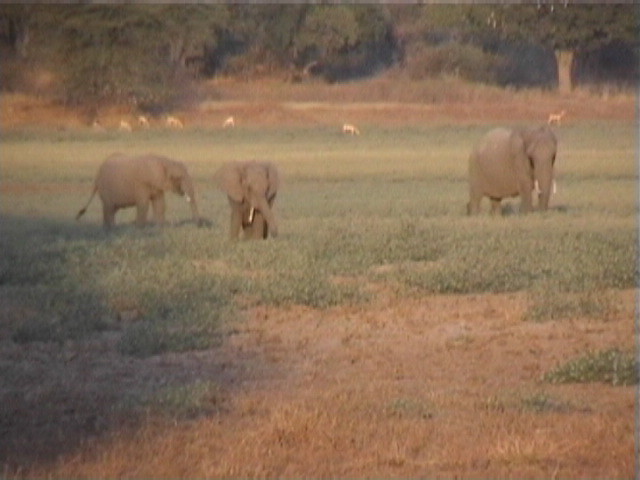In this image, taken during the late afternoon or evening in what appears to be an African meadow or savanna, we see three gray elephants standing close together amidst a field of green and patchy brown grass. The elephants are positioned with one looking to the right, one facing forward in the center, and another also facing forward to the right. In the background, the field extends to dense greenery with several tall green trees, one featuring a distinct brown trunk. Scattered throughout the back are smaller, indistinct animals that resemble deer or small dogs. The overall scene has a blurry, vintage quality, capturing the serene movement of the elephants grazing under the setting sunlight.